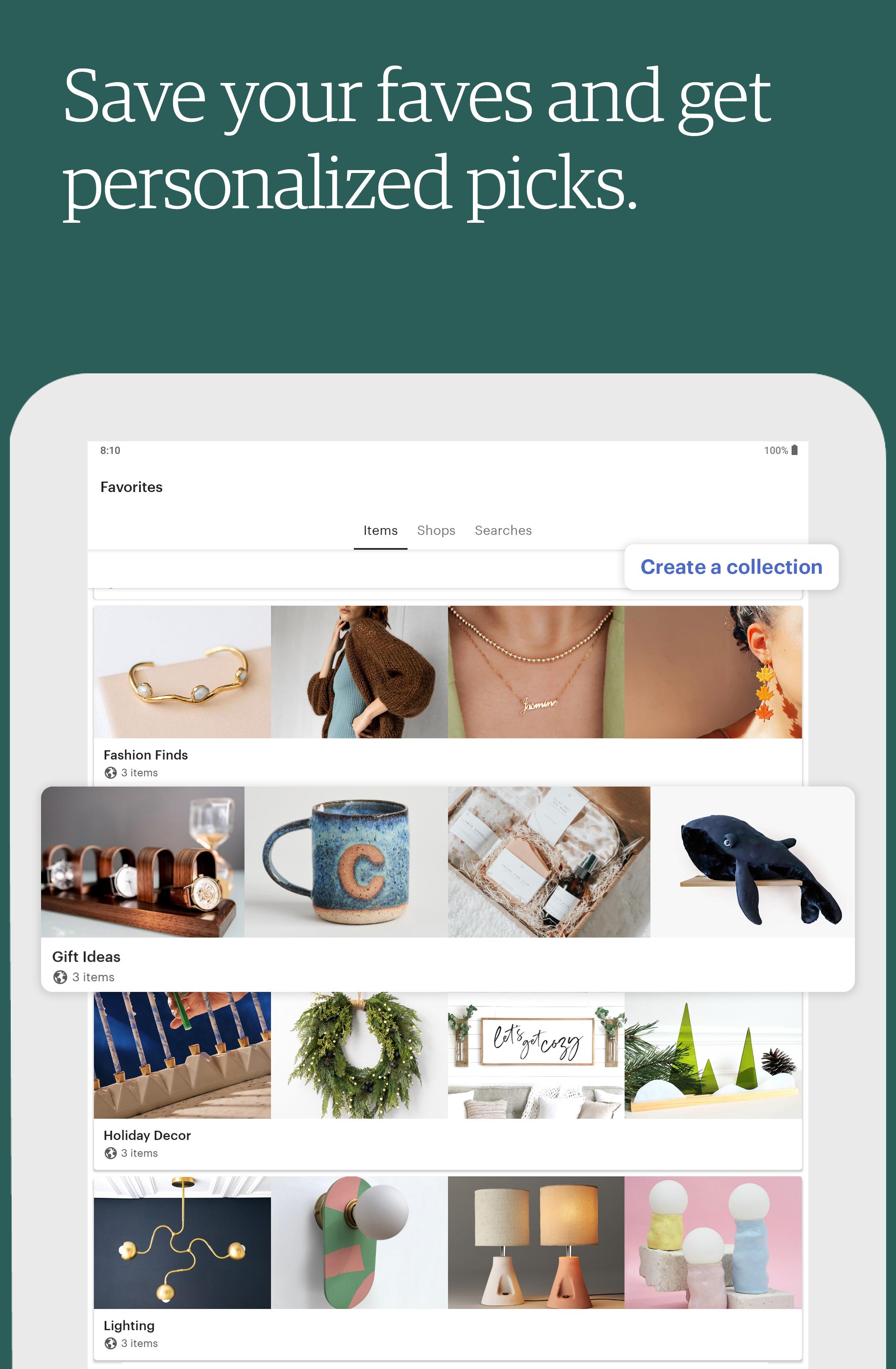The image features a dark greenish-gray background with prominent white text at the top that reads, "Save your faves and get personalized picks." Below the text, a gray box displays the options "Favorites," "Items," "Shop," and "Searches." Within this box, there's a prompt that says, "Create a Collection." Underneath the box, a detailed layout of 16 photographs is organized into four rows of four images each.

Starting from the top left:
1. A bracelet displayed prominently.
2. A model wearing a burgundy coat.
3. A necklace worn around someone's neck, seemingly made of gold.
4. A pair of earrings with yellow, orange, and red circles dangling at the bottom.

Moving to the second row:
1. A wine glass.
2. An unidentified stand.
3. A blue coffee mug with the letter "C" emblazoned on its side.
4. A collection of candy treats.

In the third row:
1. A toy whale, likely a stuffed animal.
2. A Christmas wreath.
3. A door handle.

The remaining slots in the grid are filled with various random items, enhancing the sense of variety and personalization tied to the theme of saving favorites and getting customized recommendations.